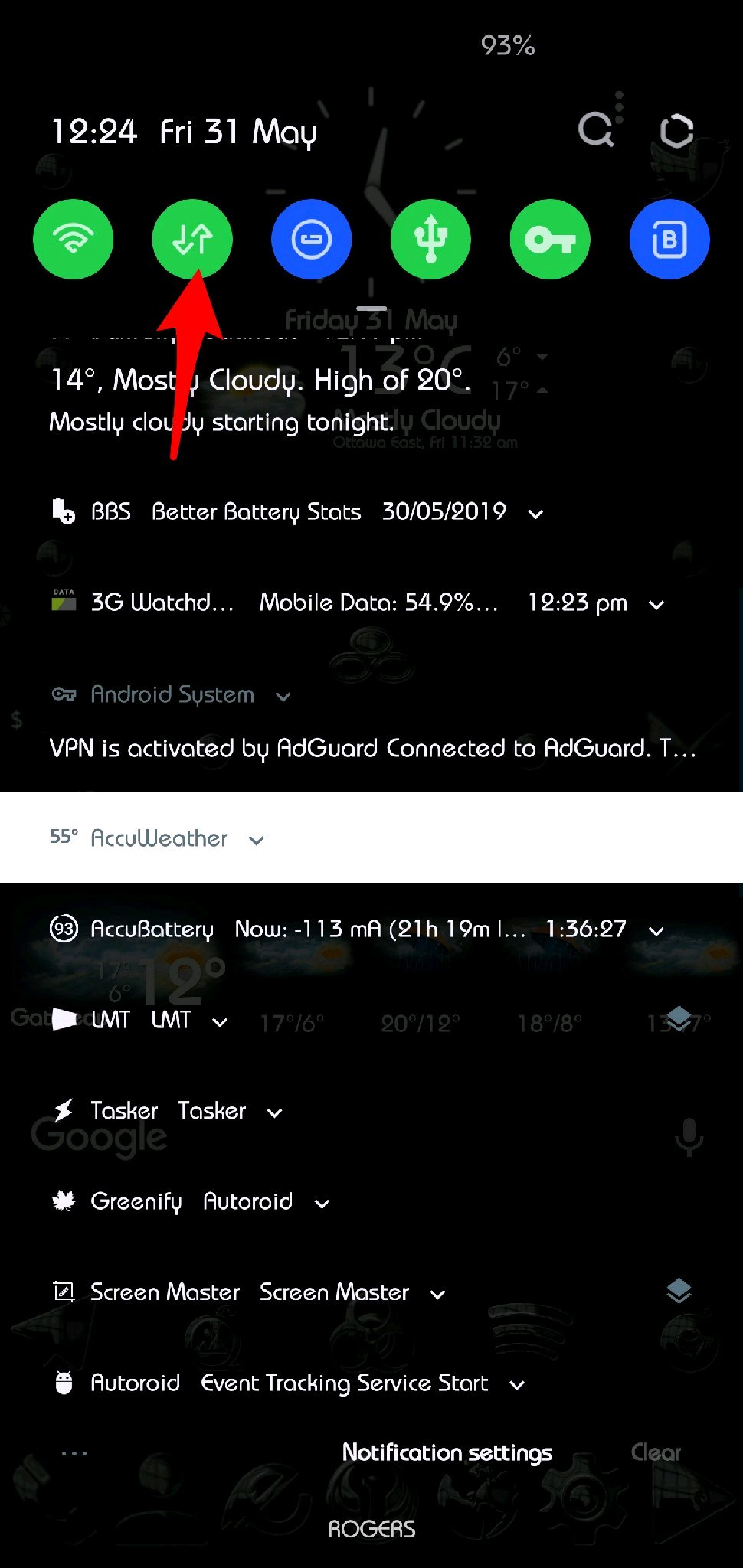This is a detailed and cleanly formulated caption for the described image:

---

The image displays two black rectangles against a black background. On the right-hand side rectangle, white text reads "93%" at the top, followed by the date format "12:24 FRI," indicating Friday, 31 May. Below this, there are six circles in total: four green and two blue. 

- The first green circle contains a Wi-Fi icon.
- The second green circle shows a white arrow pointing up and down, with a red arrow drawn next to it for emphasis.
- The third circle, which is blue, contains a white circle icon.
- The fourth green circle displays a pitchfork-like symbol.
- The fifth green circle has a white key icon.
- The final blue circle features a white letter "B."

Below the circles, white text indicates a temperature of "14 degrees" and mentions weather conditions such as "cloudy" and a "high of 20 degrees" with additional details obscured by an arrow. The text also mentions "BBS, better battery stats" followed by dates "30/2005/2009". 

Further text reads, "The VPN is activated by ADGAR, connected to ADGAR."

At the bottom of the image, more white text on a black background lists various terms and numbers: "AccuBattery now 113 mA, 21H19M, 1:36:27 LMT LMT, Taxa taxa, Greenify, Auto void, Screen master, Event tracking service, Start notification settings, Roger."

---

This caption maintains all the details from the original description while organizing the information for clarity and readability.